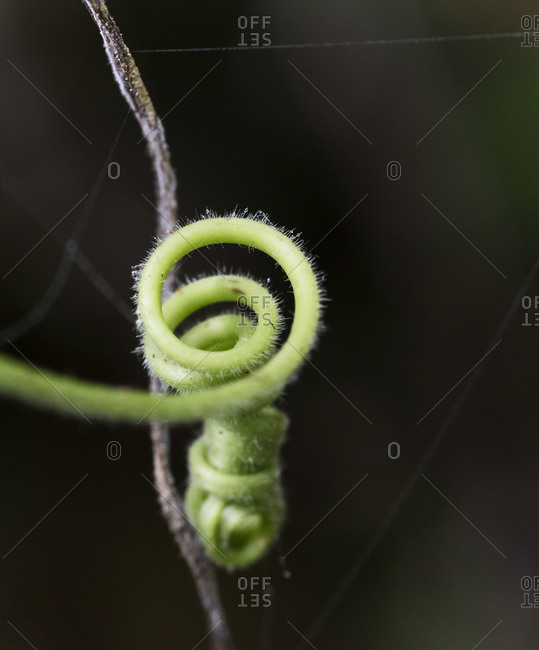The image presents a close-up view of a small green vine tendril, intricately curled around a thin, dark brown stick. The vine, light green in color, spirals and loops in a manner reminiscent of a coiled spring or a curly reptile tail. This delicate structure is covered in fine, white, hair-like filaments, which aid in gripping surfaces as it grows. The central vine tendril is the focal point, standing out sharply against a blurred background composed of green, black, and gray hues. The backdrop is predominantly dark and out of focus, enhancing the prominence of the vine. A white, diamond-shaped pattern overlay, adorned with the words "zero" and "offset," spans the top and front of the image, signaling a possible digital watermark. The stick, off to the side, runs vertically from the bottom to the top of the image, further framing the central spiraled vine.